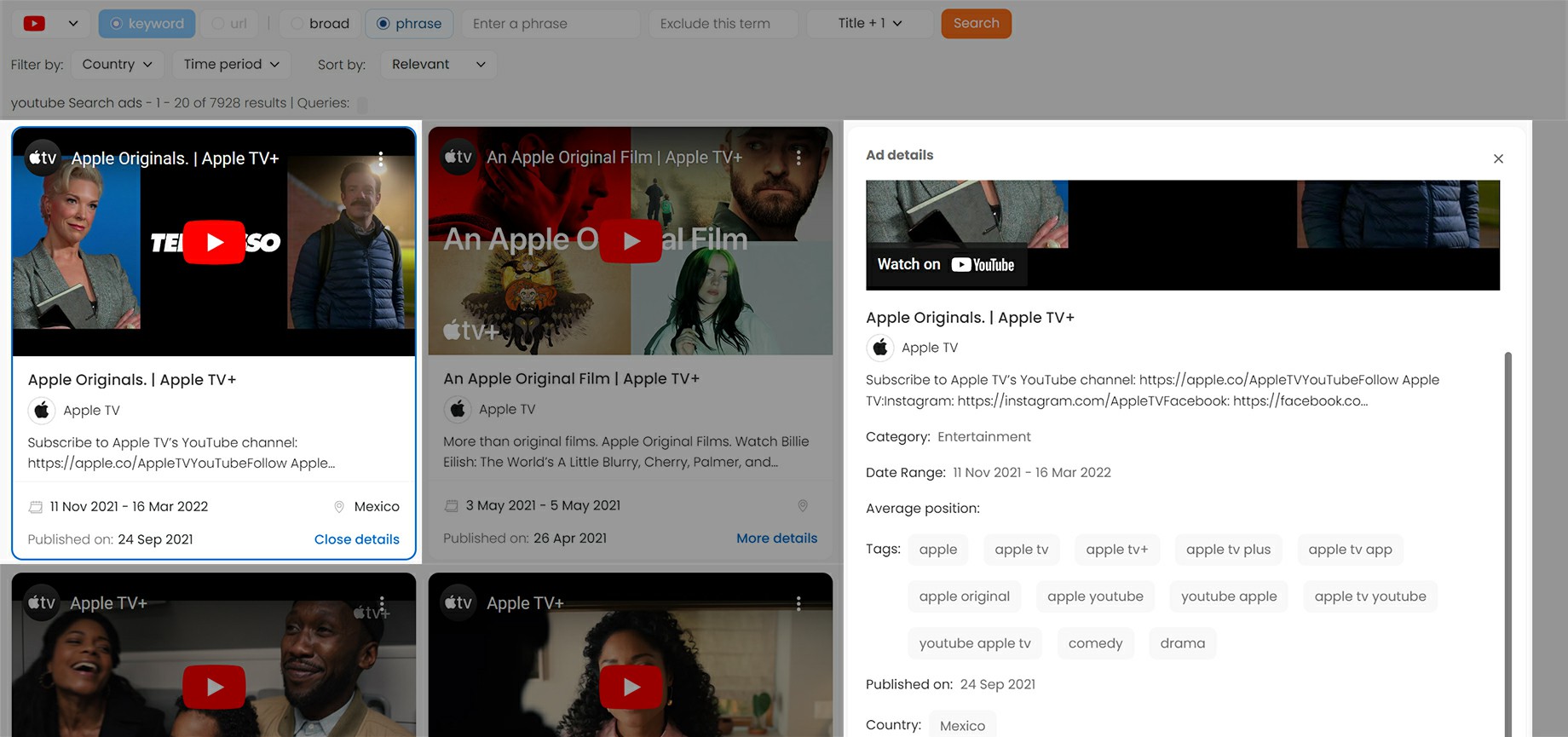**Detailed Caption for YouTube Web Page Screenshot**

The image is a partial screenshot of a YouTube web page, showcasing the interface and content related to Apple TV+. At the top of the page is the YouTube logo along with a drop-down arrow and a keyword search box. Below, there are several filter options including "Enter a phrase," "Exclude this term," "Country," "Time period," and sorting by relevance. 

The primary area of the screen displays a series of YouTube videos focused on Apple TV+ originals, recognizable by the prominent Apple logo and video thumbnails featuring actors. The highlighted video is an official Apple TV+ promotional video, titled "Apple Originals | Apple TV+", which features an invitation to subscribe to the Apple TV YouTube channel, alongside a link to the Apple website (http://apple.com/apple-tv/). 

The information panel for the highlighted video provides detailed metadata including timestamps from "11 November 2021 to 16 March 2022," with the video's publishing date marked as "24 September 2021" and the location set to "Mexico." There is an option to close this detailed section.

Following the highlighted video, three additional video thumbnails and their accompanying details are visible. Each belongs to the "Entertainment" category, share the same publish date ("24 September 2021"), and are tagged with keywords such as "Apple," "Apple TV," "Apple TV Plus," "Apple TV app," "Apple Originals," "Apple YouTube," "YouTube Apple TV," "Comedy," and "Drama." The country of origin for these videos is also "Mexico." 

Overall, this screenshot provides a glimpse into the YouTube channel dedicated to Apple TV+, featuring curated content and various filtering options for an enhanced user experience.